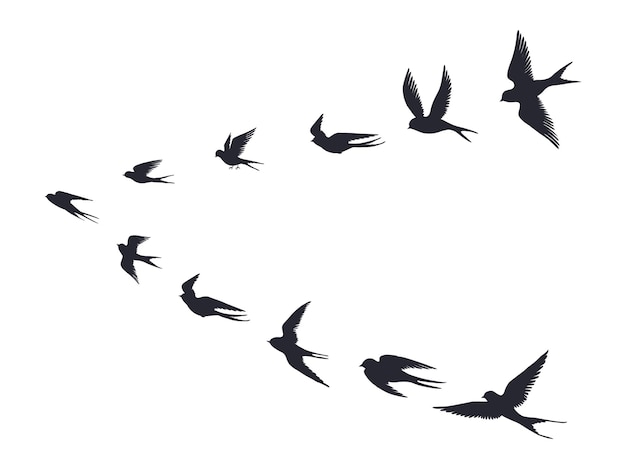This image depicts a flock of 11 birds flying in a V formation against a stark white background. The formation consists of five birds on either side of a central bird at the point of the V, all heading toward the left. These birds are represented as black or very dark brown silhouettes, emphasizing their uniformity and collective movement. Each bird’s wings are in various stages of flight: the two birds at the wider part of the V have their wings fully outstretched, showcasing the broad span of their wings and tail feathers. Other birds have their wings positioned either above, behind, or tucked in, particularly the leading bird, which gives the impression of dynamic flight. This V formation not only illustrates the aerodynamic efficiency the birds achieve by flying this way but also symbolizes cooperation and mutual support within the group.